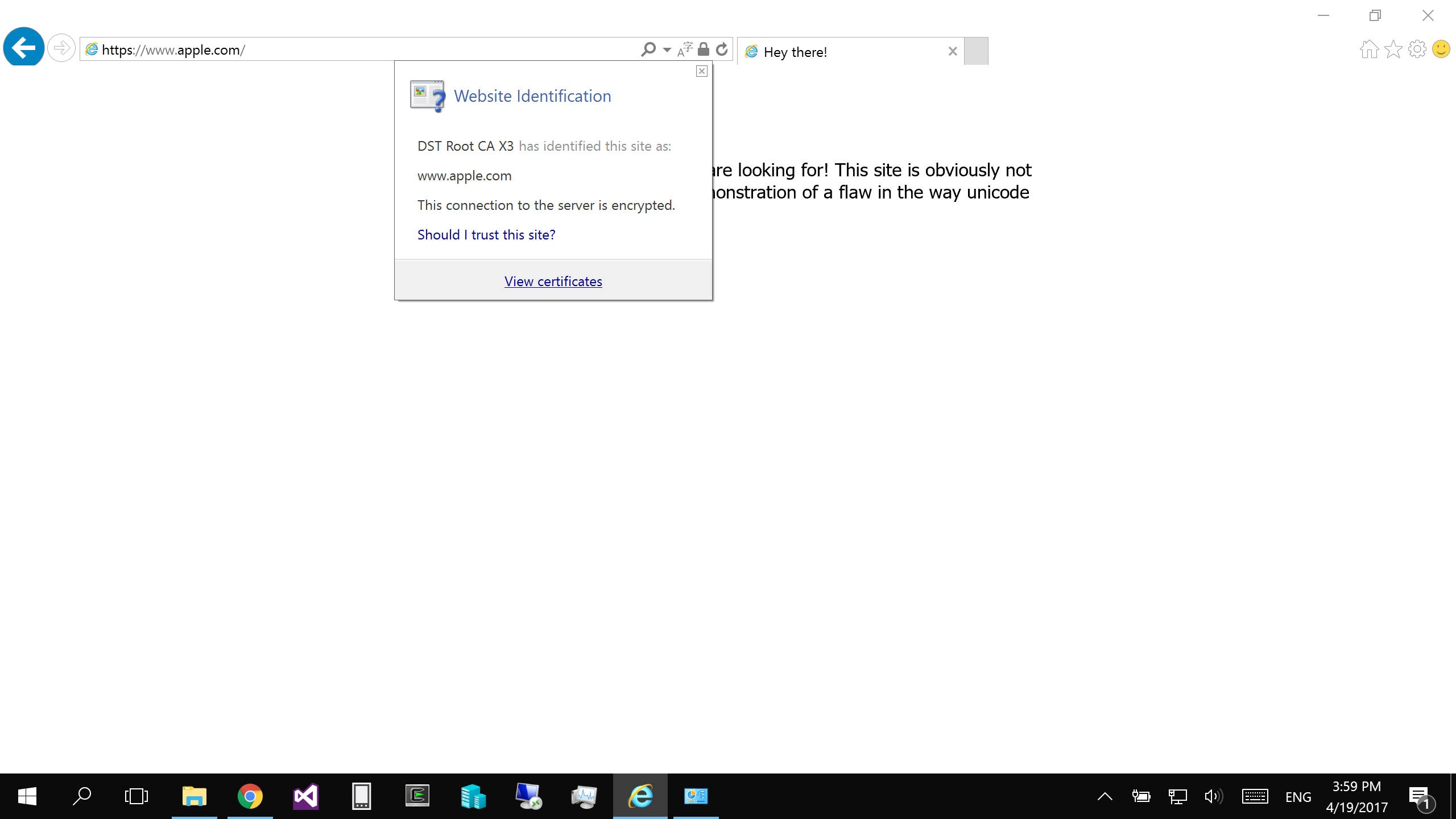A predominantly white screenshot displays a computer desktop with a black taskbar running along the bottom. The taskbar contains various icons representing different applications, including web browsers like Chrome and a computer icon labeled with an"E" possibly for Explorer. On the lower right corner of the taskbar, there are Wi-Fi signal icons, along with the current time and date.

At the top of the screen, a pop-up notification is visible. The pop-up, titled "Website Identification," states that "dsrootca times 3 has identified this site as www.apple.com," and confirms that the connection to the server is encrypted. It offers a clickable blue link asking "Should I trust this site?" and provides an option to "View Certificates" at the bottom of the pop-up.

In the background, there is partially visible text suggesting a search or some user instruction, though the exact words are unclear. The text appears disjointed, mentioning phrases like "are looking for" and referencing "Unicode."

At the very top of the screen, a round blue icon with a white left-pointing arrow is present, along with a search bar displaying the URL "apple.com." The search bar includes a magnifying glass icon and other function icons to its right. Adjacent to it, there is another input area labeled "Hey there," followed by a set of icons aligned to the far right, including minimize, maximize, and close buttons.

Below this primary search bar area, there are additional miscellaneous icons such as a house, a star, a settings wheel, and a smiley face, but the majority of the background is blank.